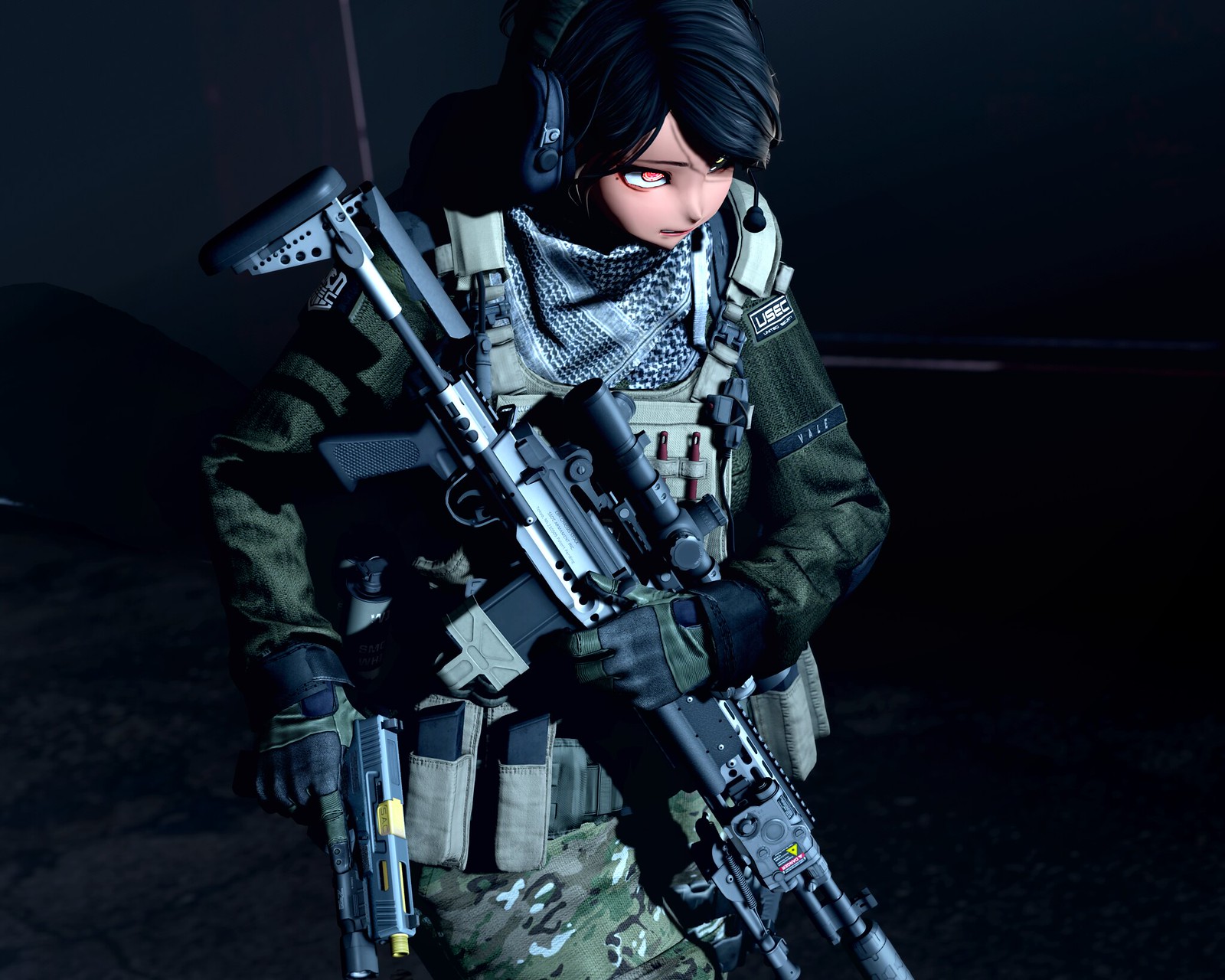In the center of the image, a digitally created female soldier stands firmly indoors in a dimly lit, war-torn setting, with hints of a stone floor partially visible and an overall dark black backdrop. She has striking black hair and intense pink eyes, a detail that emphasizes her anime-like features. She is dressed in a comprehensive military outfit with a navy green (or possibly army green) jacket and camouflage pants. A tactical headset, complete with a microphone positioned at her mouth, adorns her head. 

Her ensemble includes a bulletproof vest loaded with extra ammunition, including multiple magazines and possibly other items like knives or small tools. The vest pockets across her chest are brimming with gear, and another belt around her hips carries additional bullets and possibly more equipment. She holds a large gun strapped across her chest, likely a sniper rifle given its size, while her right hand is on a pistol holstered at her waist. The atmosphere suggests a high-stakes environment typically found in a military zone in video games, with no text visible anywhere in the image. The prominent colors include black, various shades of green, gray, white, tan, brown, red, and orange, adding to the gritty feel of the scene.